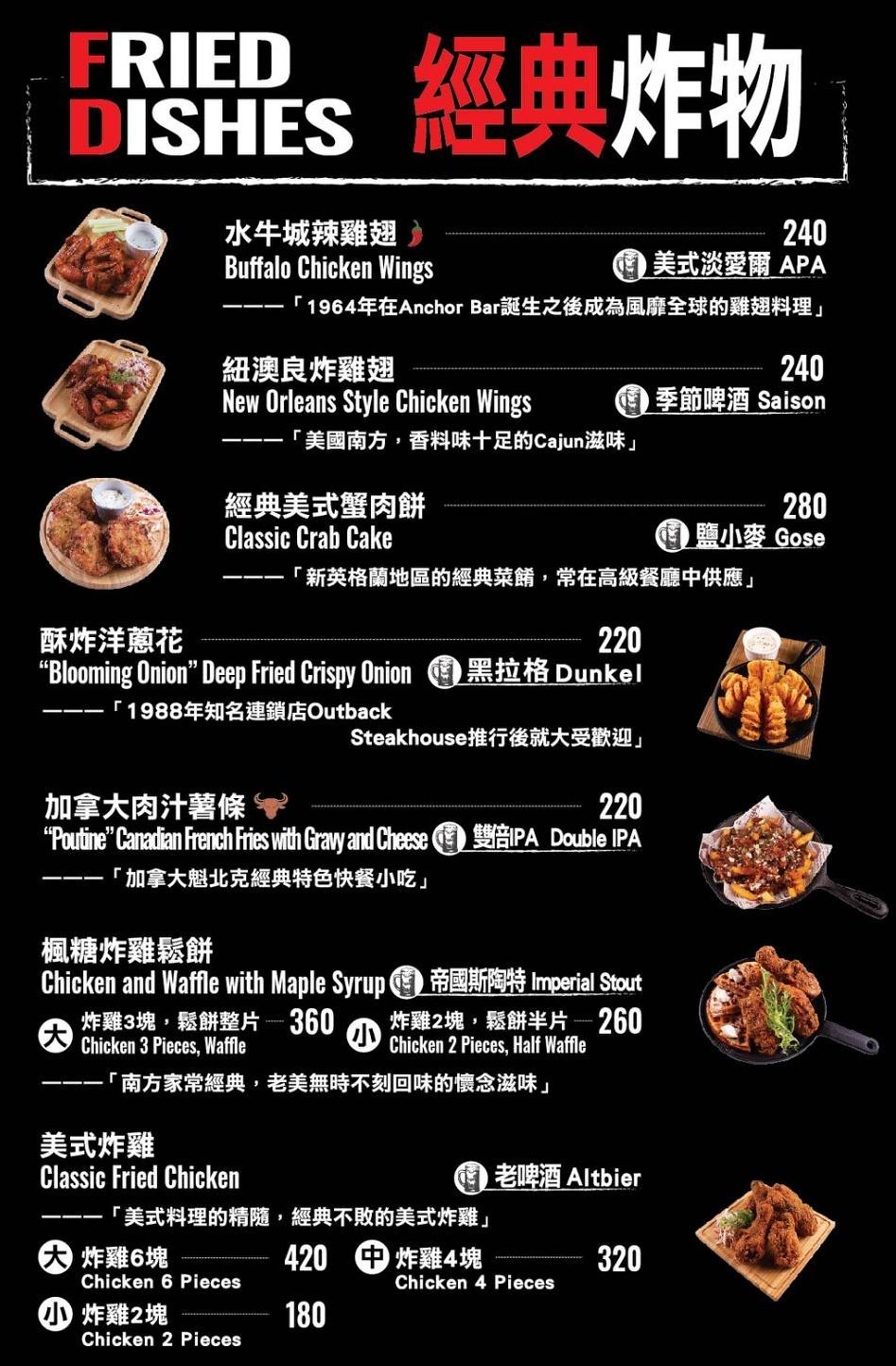This is an image of a visually striking menu page, predominantly featuring a Japanese-inspired aesthetic with its content in Japanese kanji and English. The color scheme is primarily black, white, and red. The background is black, with white text and red highlights for emphasis. 

At the top of the page, the header reads "Fried Dishes," with the 'F' and 'D' in red, while the rest of the letters are in white. Below this title, the equivalent Japanese kanji characters mirror the color scheme, with the initial characters in red.

The menu lists several delectable options, each accompanied by vivid images of the dishes:

1. **Buffalo Chicken Wings** - Priced at $2.40, presented in a wooden tray, served with sauce and celery sticks.
2. **New Orleans Style Chicken Wings** - Served in a similar rustic wooden tray.
3. **Classic Crab Cake** - Plated on a wooden plate, accompanied by tartar sauce and coleslaw.
4. **Blooming Onion** - Modeled after the iconic dish from Outback Steakhouse, this fried onion is served in a cast iron skillet, its petals arranged in an appealing mountain-like pattern.
5. **Poutine** - A Canadian specialty featuring French fries, gravy, and cheese, also served in a cast iron skillet.
6. **Chicken and Waffles** - A sweet and savory classic, served with maple syrup in a cast iron skillet.
7. **Classic Fried Chicken** - Displayed on a square plate, showcasing its golden, crispy exterior.

The layout and presentation of the dishes, placed on wooden trays or cast iron skillets, add a rustic charm, complementing the menu's sophisticated yet simple design.